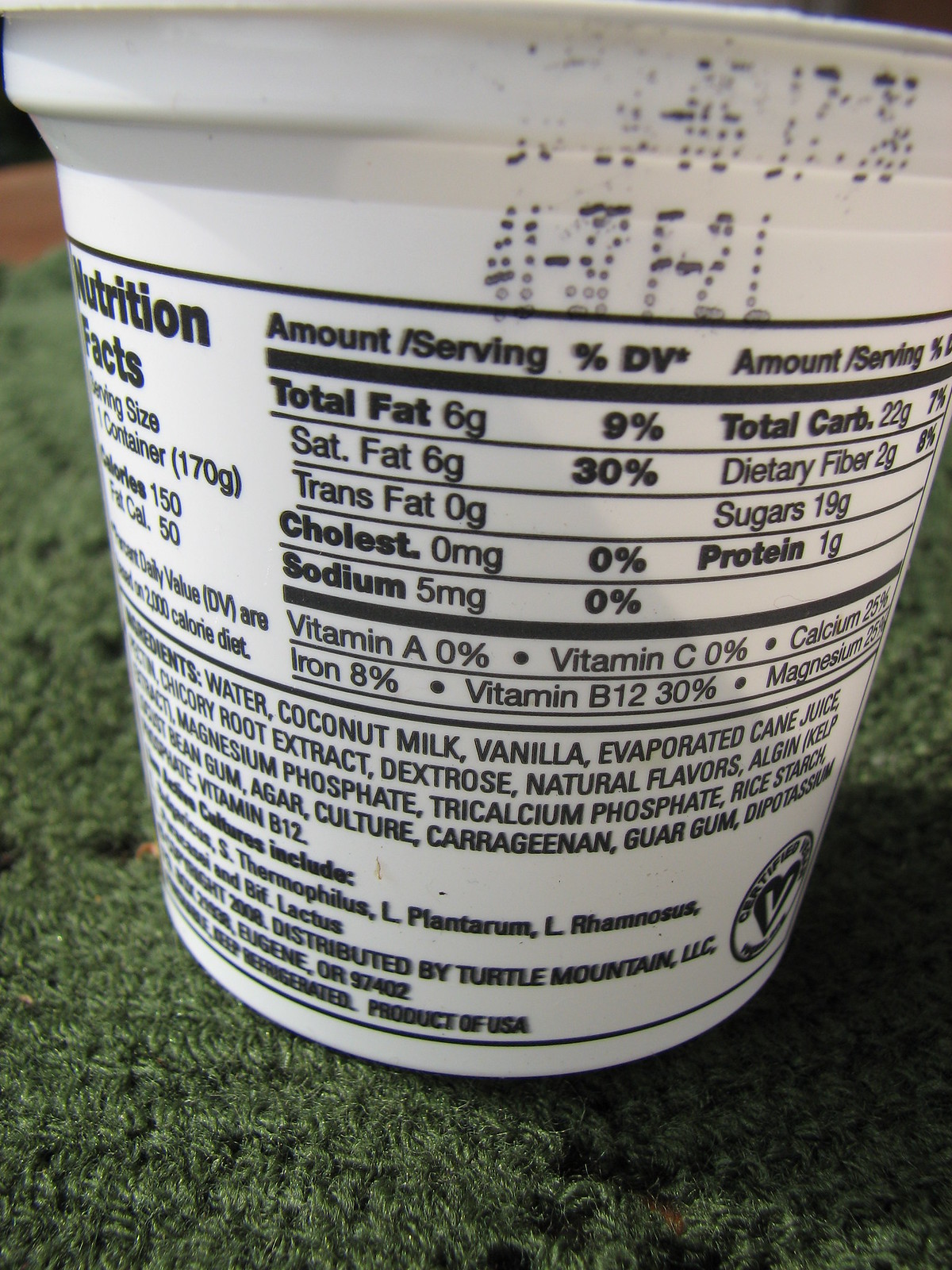This close-up photograph captures a container of yogurt placed against a vivid green tablecloth backdrop. The image focuses intently on the nutritional information and ingredient list, presenting a clear and detailed view. The yogurt's serving size is noted as one container, weighing 170 grams and delivering 150 calories, with 50 calories derived from fat. It contains 6 grams of total fat, all of which is saturated fat, with no cholesterol. The sodium content is minimal at 5 milligrams. Carbohydrates total 22 grams, including an admirable 2 grams of dietary fiber but a high 19 grams of sugar. Protein content is low, at just 1 gram. Below the nutritional facts, the ingredient list is also visible, though not legible in this description. The text is printed in a straightforward, easily readable format, ensuring that important dietary information is readily accessible to consumers.